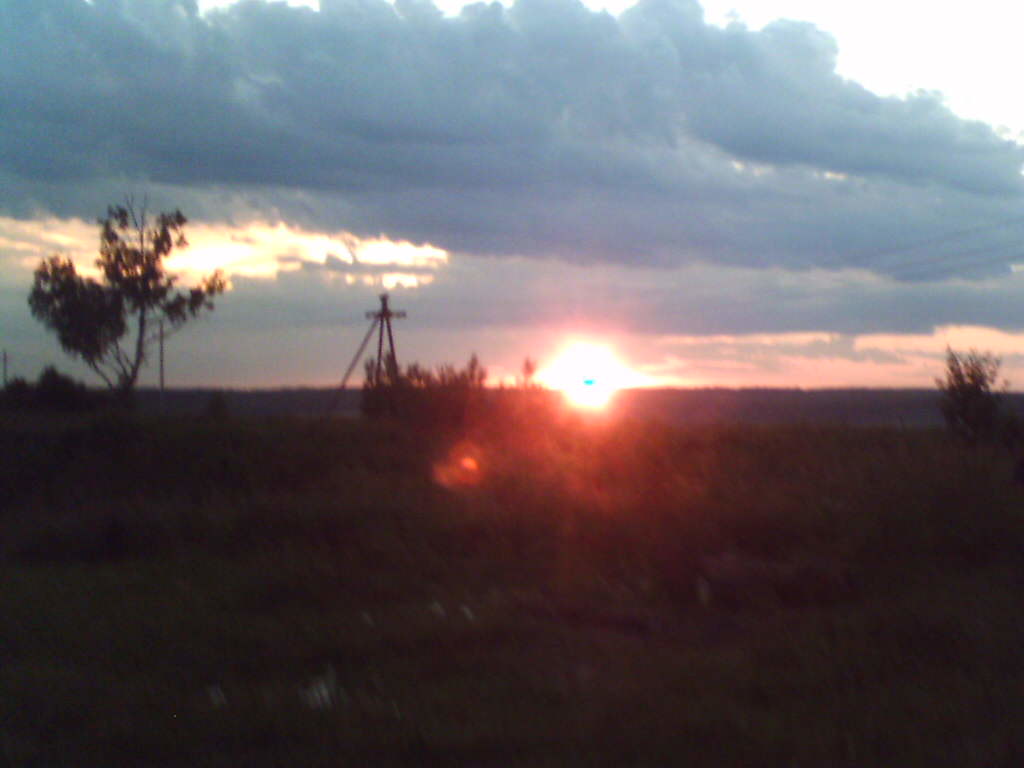In this outdoor image, we see a serene landscape at either sunrise or sunset, enveloped in a gray, cloudy sky with heavy cloud coverage. The sun, glowing brightly at the horizon, casts a reddish glare over the scene, illuminating the grassy area in the foreground. The sky's hues transition from a white at the top to an orangish shade near the horizon. The picture, slightly blurry and hazy, makes it difficult to discern specific elements in detail.

The landscape features several trees; most of them are short with sparse leaves, except for one taller tree that stands out. Additionally, there are some bushes scattered across the middle area, including the right-hand and left-hand sides. Amongst the foliage, a structure resembling an easel or possibly a pole with protrusions is visible to the left of the sun, adding an intriguing element to the scene. The ground is covered in brush, and due to the overall darkness, the colors of the foliage appear muted and indistinguishable.